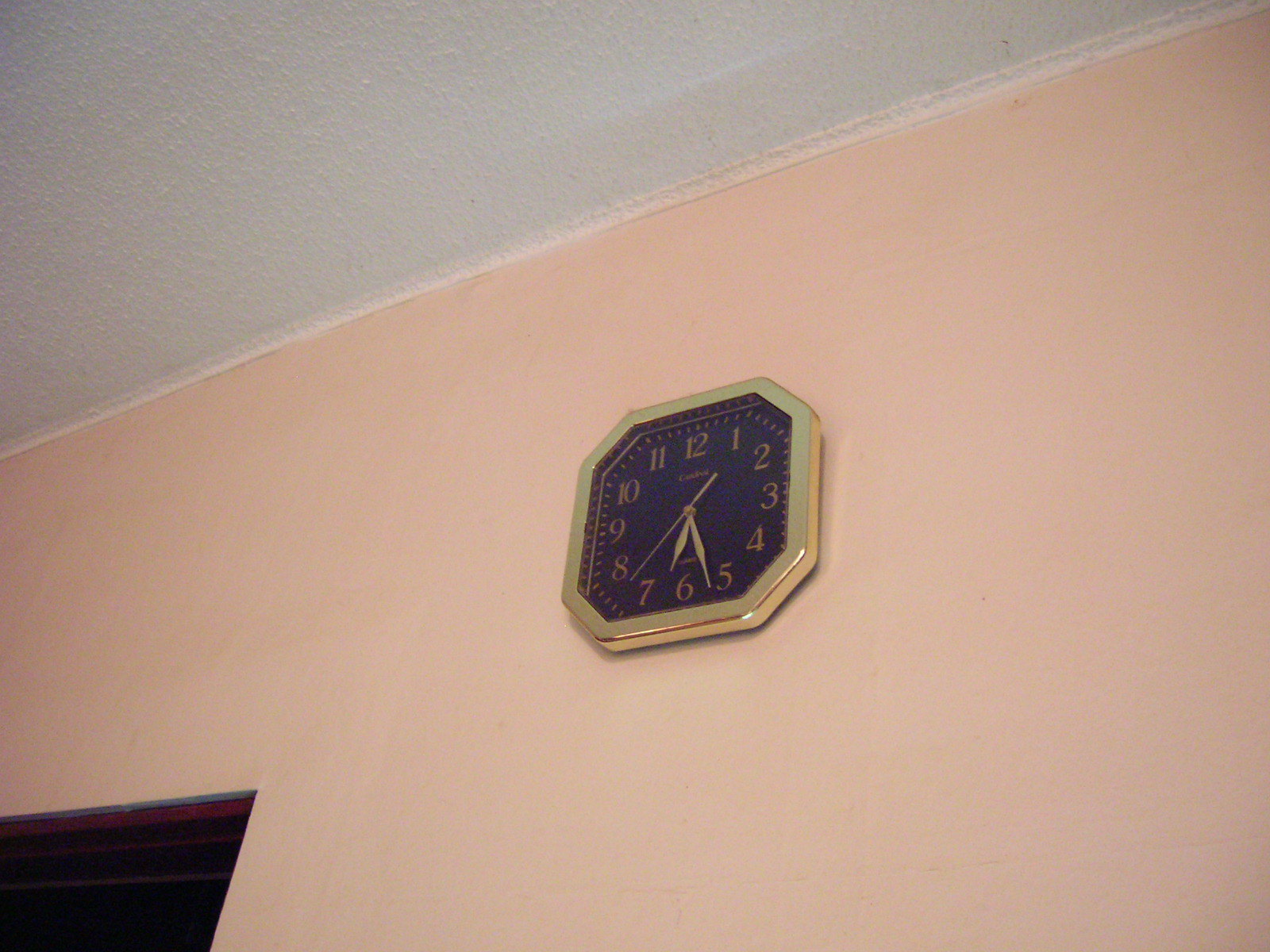This photograph showcases a vintage wall clock adorned with a gold bezel featuring an octagonal shape, although it can also be interpreted as a hexagon due to its configuration of four main sides and four smaller sides, with distinct corners. The clock's face is black, providing a striking contrast to the gold bezel. It boasts a classic analog dial with elegant second, minute, and hour hands. This timepiece, reminiscent of the aesthetic styles of the 1980s and 1990s, hangs on a peach-colored wall beneath a textured ceiling. In the lower left corner of the image, there is a doorway that slightly intrudes into the frame, adding to the vintage ambiance of the setting.